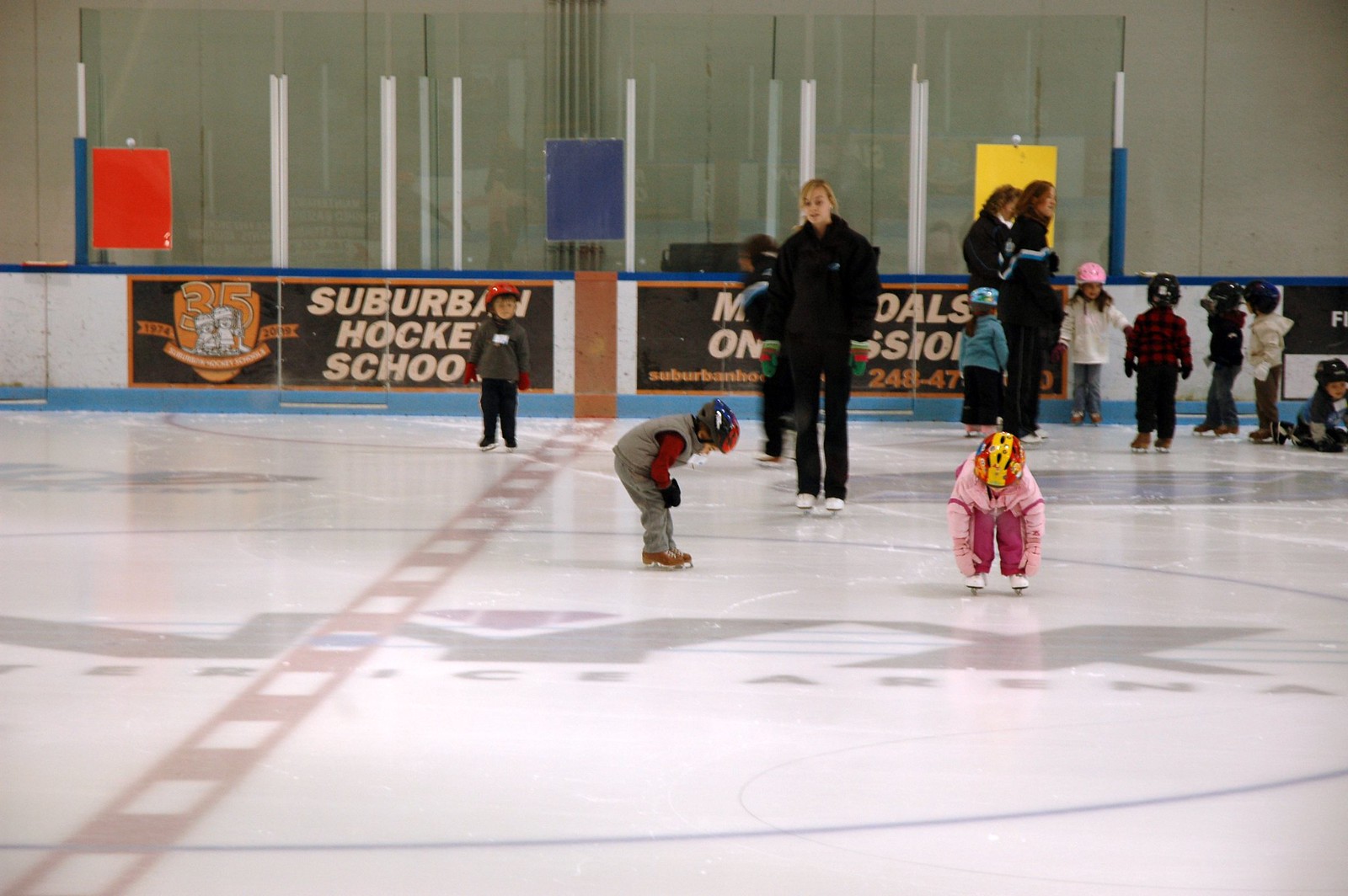The image depicts a scene at a hockey rink primarily used for teaching skating to children. Approximately 10 small children are equipped with ice skates, helmets, protective gear, and warm clothing, standing or cautiously moving on the ice. In the foreground, two children are bending forward as if attempting to skate, while others in the background are lined up against the side wall of the rink. Three adults are present, overseeing and presumably conducting the skating lessons. The rink itself is predominantly white with elements of red and black visible through the ice. The surrounding wall of the rink features a blue trim at the bottom, glass panes with metallic posts above, and various banners at the top. One prominent banner reads "Suburban Hockey School" in bold white and orange letters on a black and orange background. Further beyond the glass panes, the actual facility walls are a white color, highlighted by the vibrant activity on the ice.